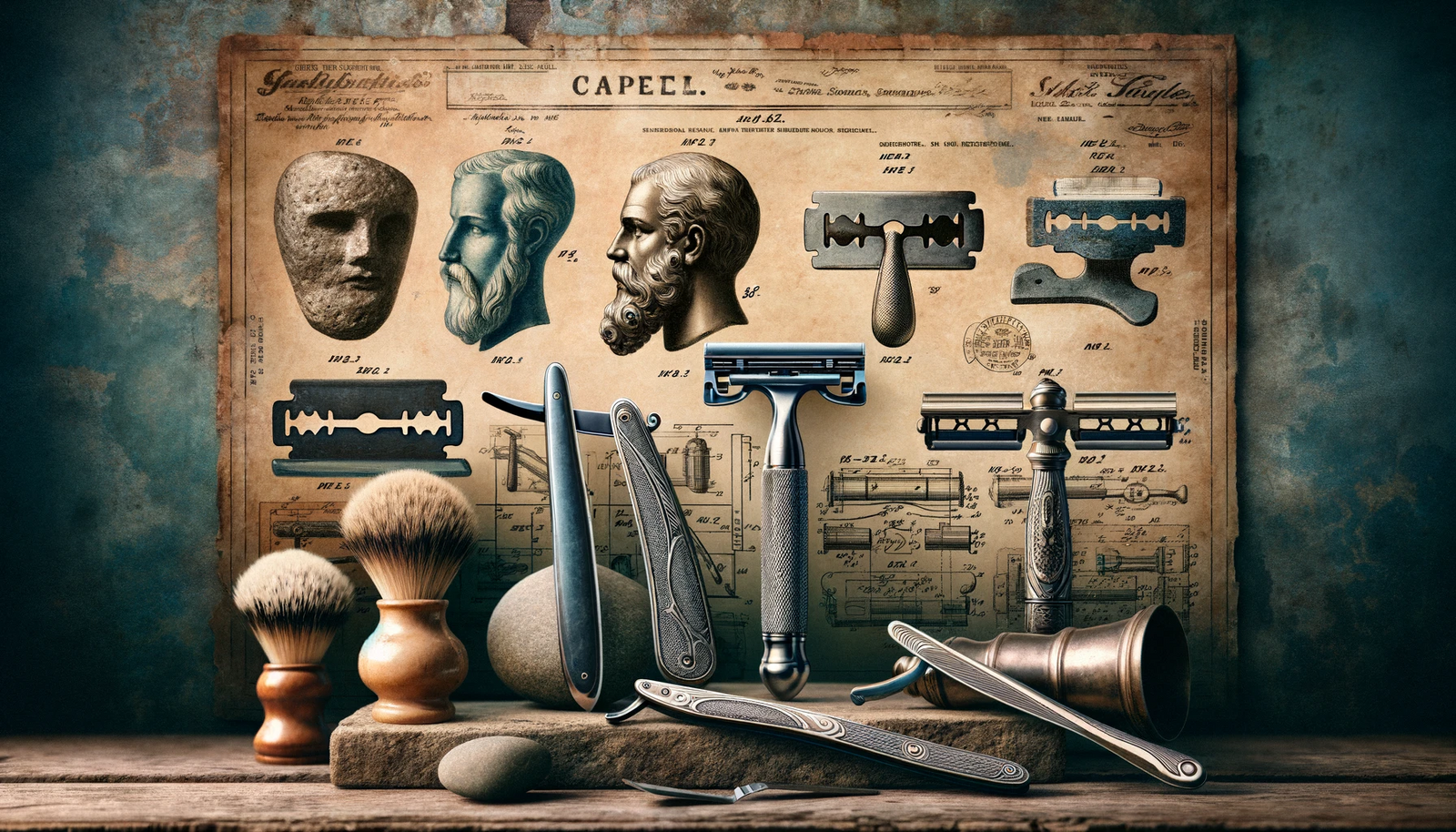In this digital illustration, an old, outdated poster is displayed prominently on a dark blue and beige wall. The poster, printed on aged brown paper, features an antiquated font and showcases three statue heads on the left side: one faceless, another of a bearded man in a blue-gray hue, and a similar bearded figure in a bronze finish. On the right side of the poster, metal tools resembling scrapers or ancient shavers are depicted. Below the poster, sitting on a wooden bench or table, is a collection of historical grooming tools, including two brushes, various blades, razors, and potentially knives. The overall theme suggests a glimpse into the historic practices of shaving and grooming, with elements that highlight the evolution of such tools over time.